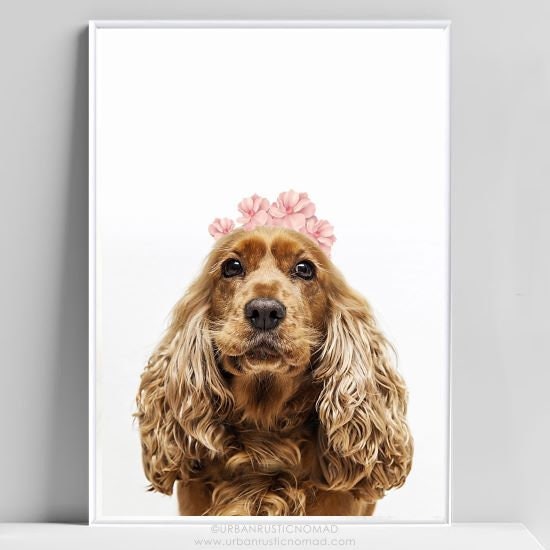In this highly detailed image, we have a framed photograph, not a painting, set against a gray wall. The frame is white, medium-sized, and houses a large, printed photograph of a charming Cocker Spaniel. The dog, showcasing luxuriant, long and curly ears that cascade down its sides, features predominantly light brown fur with a spot of white on its muzzle and some speckles of brown on its black nose. Its expressive brown eyes gaze directly at the viewer, exuding a joyful and expectant demeanor, amplified by a slight, whimsical grin and a half-open mouth. Adorning the dog's head is a delicate tiara made from four small pink flowers, arranged to form a floral crown, adding to its endearing appearance. The bottom of the photograph includes faint, difficult-to-read gray text that states, "© Urban Rustic Nomad www.urbanrusticnomad.com." The high realism of the photo almost blurs the line between a detailed painting and a photograph, capturing the essence of this adorable pet with photographic precision.